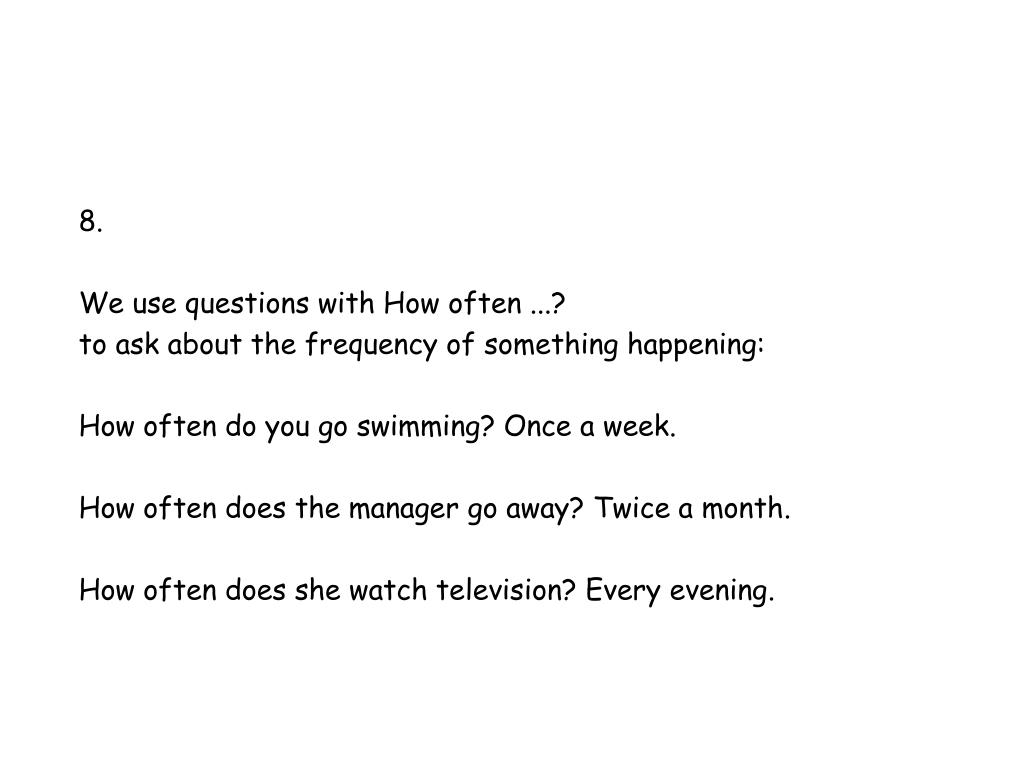The image features a minimalistic, all-white background with black text in a casual, unidentified font. At the top left corner, the number "8." is prominently displayed. Below this numeral, the text instructs on the usage of "how often...?" questions to inquire about the frequency of various activities, followed by a colon:

**"How often...?" to ask about the frequency of something happening:**

A blank line separates this introductory text from the subsequent examples:

1. **Example Question:** "How often do you go swimming?"
   **Response:** "Once a week."

2. **Example Question:** "How often does the manager go away?"
   **Response:** "Twice a month."

3. **Example Question:** "How often does she watch television?"
   **Response:** "Every evening."

The image serves as a simple instructional guide on forming questions regarding the regularity of actions, with clear examples and corresponding responses.